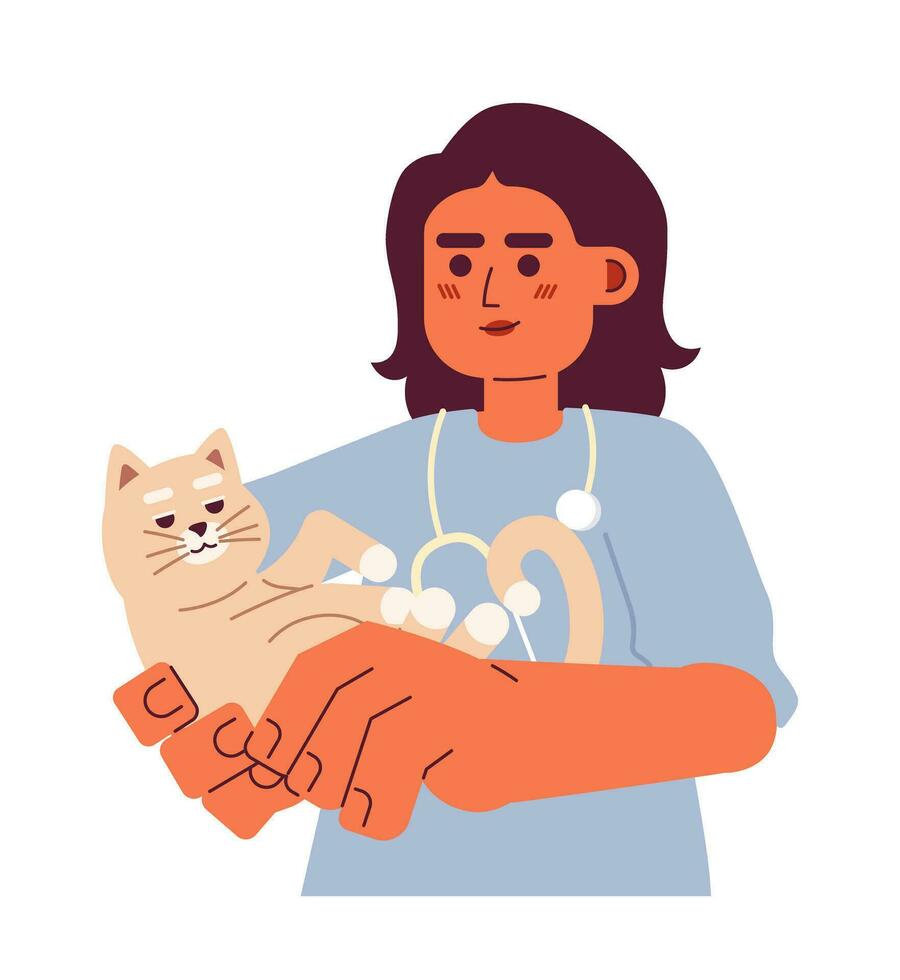The image is a stylized, comic book-like hand illustration of a female veterinarian, likely intended for veterinary service promotions. The woman has a tan complexion and dark, shoulder-length hair, suggesting she might be of Hispanic descent. She wears a light blue scrub top and has a stethoscope around her neck. Notably, her hands are exaggeratedly large, a result of the foreshortening effect, extending toward the viewer as she holds a tan-colored cat. The cat, which has white paws, white-tipped tail, brown eyes, brown nose, and white eyebrows, lies on its back with a pleasant, content expression. It looks directly at the viewer, with its three whiskers on each side of its nose clearly visible. The veterinarian holds the cat away from her body, emphasizing the size of her hands further and contributing to the overall whimsical, cartoonish aesthetic of the illustration.